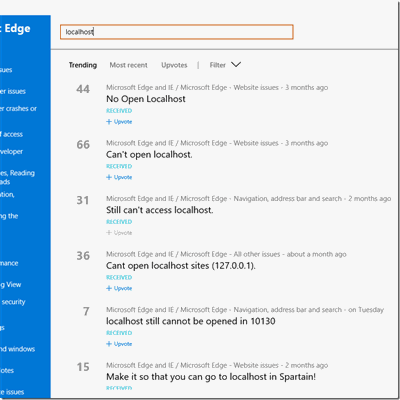**Detailed Caption:**

The image showcases an internet configuration screen on a Windows device, identifiable by the presence of Microsoft-related elements and the "Edge" label in the top left corner. The user interface shown is likely part of a desktop or laptop operating system.

At the very top of the screen, there is an orange search bar with the text "localhost" typed in. Below this search bar, there is a navigation menu with the labels "Trending," "Most Recent," "Upvotes," and "Filter," the last of which features a dropdown menu.

The main content area displays a list of issues related to accessing the localhost in Microsoft Edge and Internet Explorer (IE). There are six issues listed, each denoted by a light grey number:

1. **44** - "Microsoft Edge and IE: Website issues three months ago, no open localhost. Received. Upvote available."
2. **66** - "Can't open localhost in Microsoft Edge."
3. **31** - "Still can't access localhost."
4. **36** - "Can't open localhost sites (127.0.0.1)."
5. **7** - "Localhost still cannot be opened in 101.3.0."
6. **15** - "Make it so that you can go to localhost in Spartan."

This screen appears to be part of a compilation website where users can report error messages, share experiences, and look for potential solutions to their technical issues.